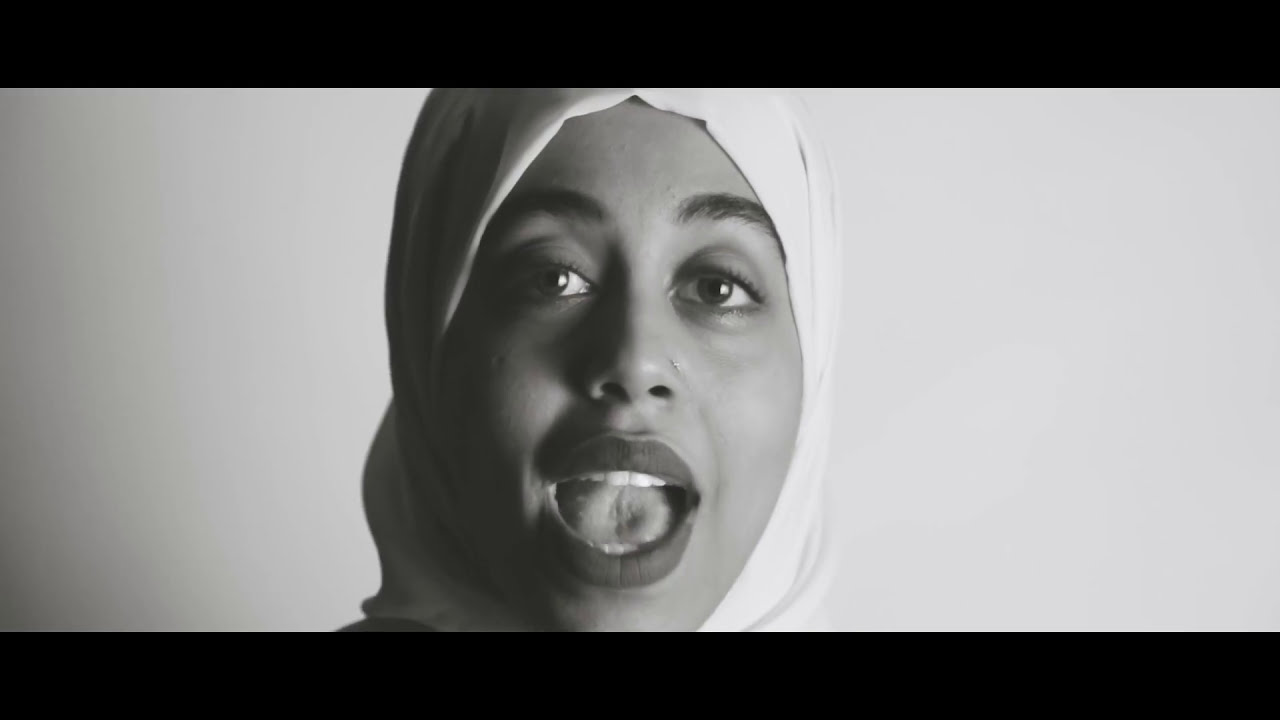The monochrome image features a close-up of a woman’s face, centered against an off-white background that darkens towards the left. She is wearing a tightly-wrapped white hijab that conceals her hair and ears, extending to chin level. Her facial features suggest she might be wearing lipstick, as indicated by the contrast of her lips. The woman’s mouth is open, revealing the top half of her front teeth and the tip of her tongue against them, expressing an emotion that could be happiness, surprise, or laughter. Her eyes, possibly brown, and dark eyebrows are clearly visible, and she has a small stud nose piercing on her left nostril. The light source illuminates the right side of her face more prominently, casting subtle shadows on the left. The image is framed by black bars at the top and bottom, creating a focused, intimate portrait.